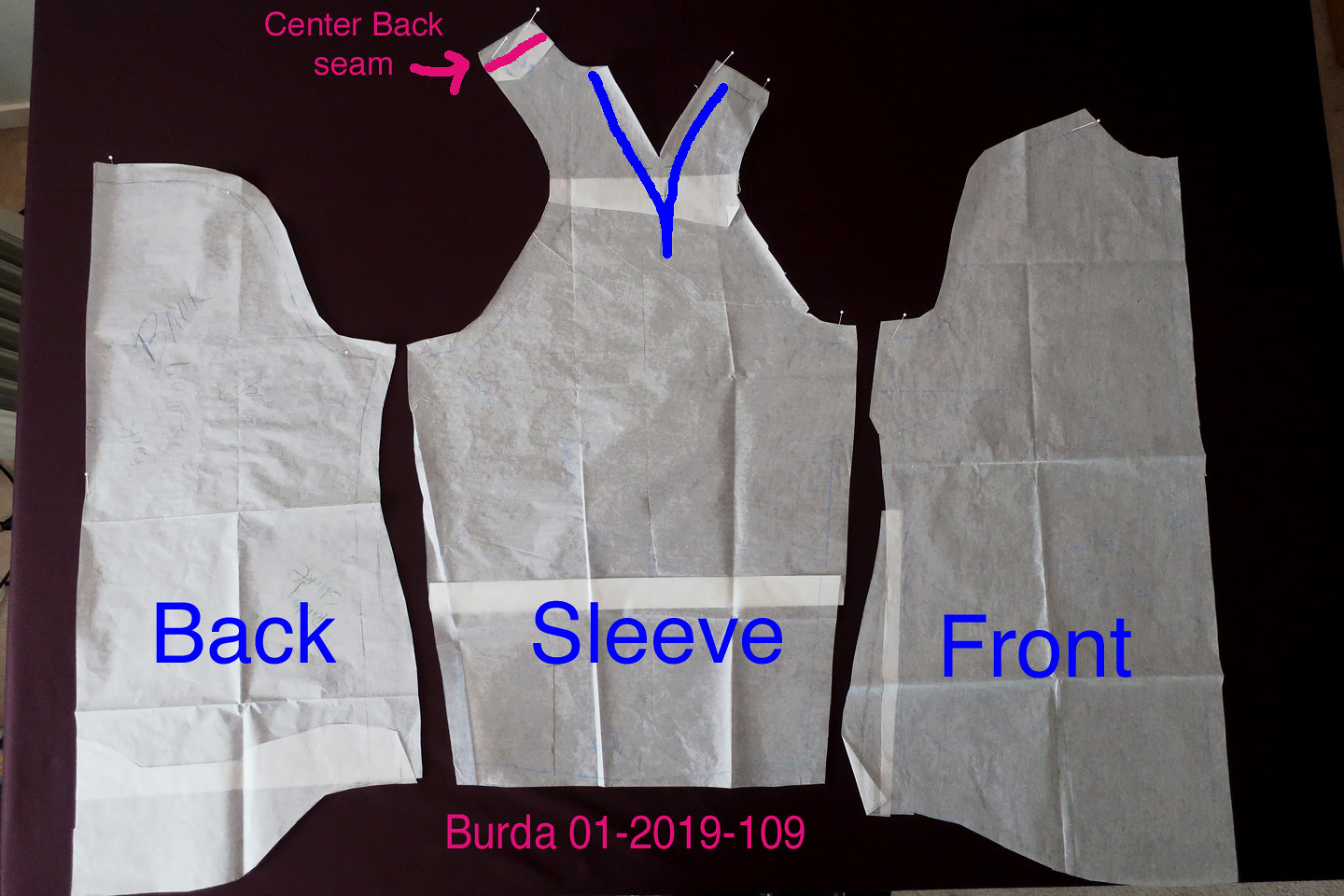The image depicts three cut-out pieces of see-through tissue paper, arranged against a black background and pinned in place. Each piece is precisely labeled in blue font. From left to right, they read "back," "sleeve," and "front." Each label highlights the function of each paper piece in garment construction. At the top, a pink inscription reads "center back seam" with an arrow pointing to the middle piece, which also features a pink line. This middle piece, labeled "sleeve," is visually distinct, resembling an apron shape with a V at the top. The left and right pieces, echoing "half an apron" forms, are indicated as "back" and "front," respectively. At the bottom center of the arrangement, the text "Berta 01-2019-109" is prominently displayed in pink.